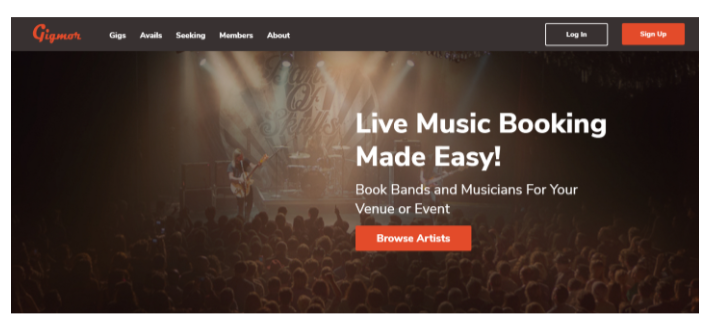In this vibrant and energetic image of the Gigmore webpage, the interface prominently displays options such as "Gigs," "Avails," "Seeking," "Members," and "About." The top right corner features buttons for "Login" and "Sign Up." The homepage tagline reads "Live Music, Music Booking Made Easy," emphasizing the platform's mission to facilitate easy booking of bands and musicians for venues or events. Users can "Browse Artists" to find the perfect fit for their needs. In the background, a lively stage scene captures a band immersed in a performance, illuminated by professional studio lights. A lead vocalist passionately sings while strumming a guitar, accompanied by a drummer, adding rhythmic beats to the electrifying atmosphere. The crowd, partially visible, adds to the dynamic and engaging ambiance of live entertainment.